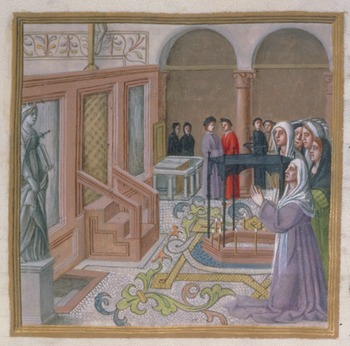This image appears to be an intricately detailed illustration, possibly from a Renaissance-era religious book, depicting a serene religious scene set inside an old, church-like building with muted pastel tones. Dominating the left side of the image is a statue of a crowned woman, likely a saint, standing regally on a podium. Several women, dressed in modest robes and with their hair covered, are gathered in front of this statue. One woman in a purple gown with a white headwrap stands prominently in prayer. To her right is a woman in green with a black shawl, and three more women can be seen nearby, all engaged in the same act of reverence. 

The marble floor underneath them boasts intricate painted details with hues of purple, red, black, and green. There is a hexagon-shaped altar near the women, emphasizing the religious context. In the background, men can be seen under high archways, divided by pinkish columns, observing the scene from a distance. These men wear fancier attire, including hats and long robes in colors like purple and red. A set of wooden stairs with railings leads up to a closed door just behind the statue. On the right side of the composition, another set of stairs and a trio of framed windows subtly enhance the architectural design. Overall, the image beautifully captures a moment of solemn devotion within a richly decorated and architecturally significant space.